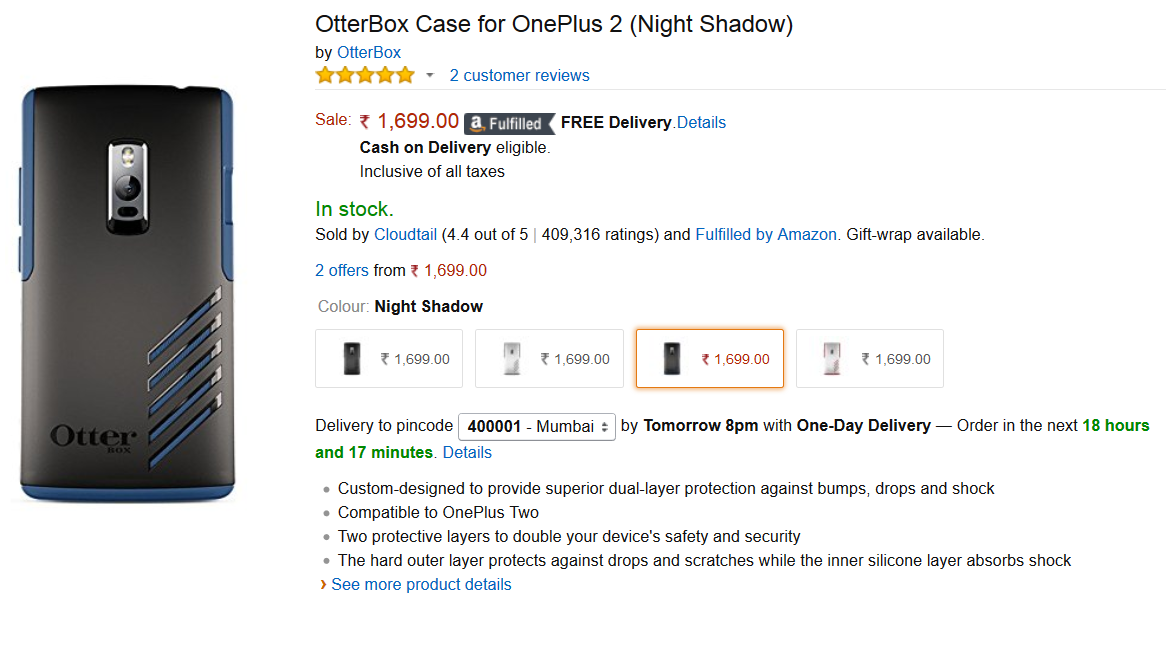**Product Listing on Amazon for Otterbox Case**

**Product:** Otterbox Case for OnePlus 2  
**Color:** Night Shadow  
**Reviews:** Rated 5 stars based on 2 reviews  
**Price:** ₹1,699 (Currency symbol not recognized, likely Indian Rupees)  
**Features:**
- Cash on delivery eligible
- Inclusive of all taxes  
**Availability:** In stock  
**Sold by:** CloudTail  
**Color Options:** Different colors available  
**Delivery Info:**  
- Delivery location: Mumbai, India
- One-day delivery available, order by tomorrow at 8 PM  
**User Interface:**
- Typical Amazon layout with a white background  
**Product Description:**
- This phone case is designed for the OnePlus 2, an Android phone. The term "1 plus 2" refers to the second-generation OnePlus phone, despite its potentially confusing naming convention.